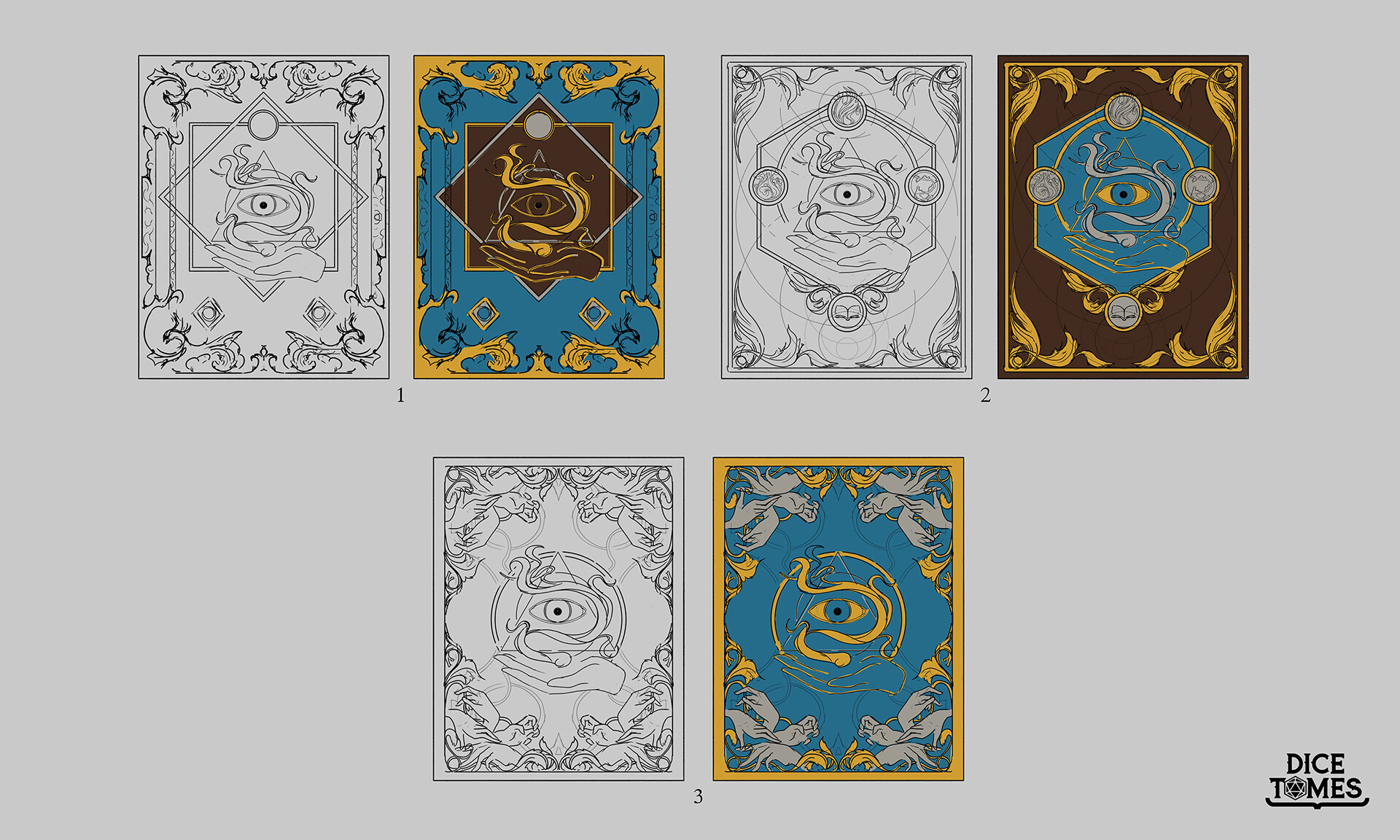This image appears to depict a series of game cards or posters, arranged in a long horizontal white rectangle with a light gray background. In the bottom right corner, the text "DICE TIMES" is prominently displayed, with the "I" creatively shaped like a multi-sided die. Below the text, a horizontal line adds emphasis.

The main content consists of six smaller rectangles, arranged in pairs, with each pair representing a numbered set labeled 1, 2, and 3. Each set includes two versions of the same abstract illustration: a black and white drawing on the left and a colored, more detailed version on the right.

Set number 1, located at the top left, features a pyramid-shaped eye held by a hand. The black and white version contrasts with the colored one which showcases a brown central eye, a blue background, and a gold border with square details.

Set number 2, situated in the middle, again features the eye in a hand but is marked by a six-sided figure surrounding the eye. The colored version has a brown background with a blue hexagon and intricate gold detailing along the edges.

Set number 3, found at the bottom, presents the eye held by a hand within a simple circular border. The colored illustration has a blue background with a gold ornate detailing and additional gray hand motifs around the edge.

The primary color scheme across the colored illustrations includes dark teal, dark brown, and gold, creating a cohesive yet intricate visual theme.